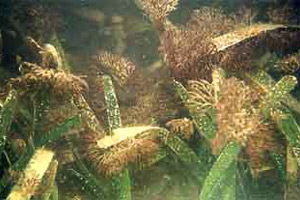The image depicts a scene that appears to be underwater, capturing a variety of plant life in what looks like a murky aquatic environment. The photo, which is somewhat low in resolution and slightly hazy, shows clusters of long, thin, green leaves interspersed with brown and yellowish foliage. The plants seem to float or sway as if suspended in water, contributing to the overall blurry and indistinct quality of the picture. In addition to the green leaves, there are branch-like structures with white and reddish tendrils, adding to the diverse underwater flora. These elements, combined with the presence of brown, possibly moss-like material and dirt, create a rich tapestry of underwater plant life that spans the image. The background has further growths of similar plants, primarily clustered on the right side, both at the top and bottom, with a smattering on the left, enhancing the view of this submerged ecosystem.